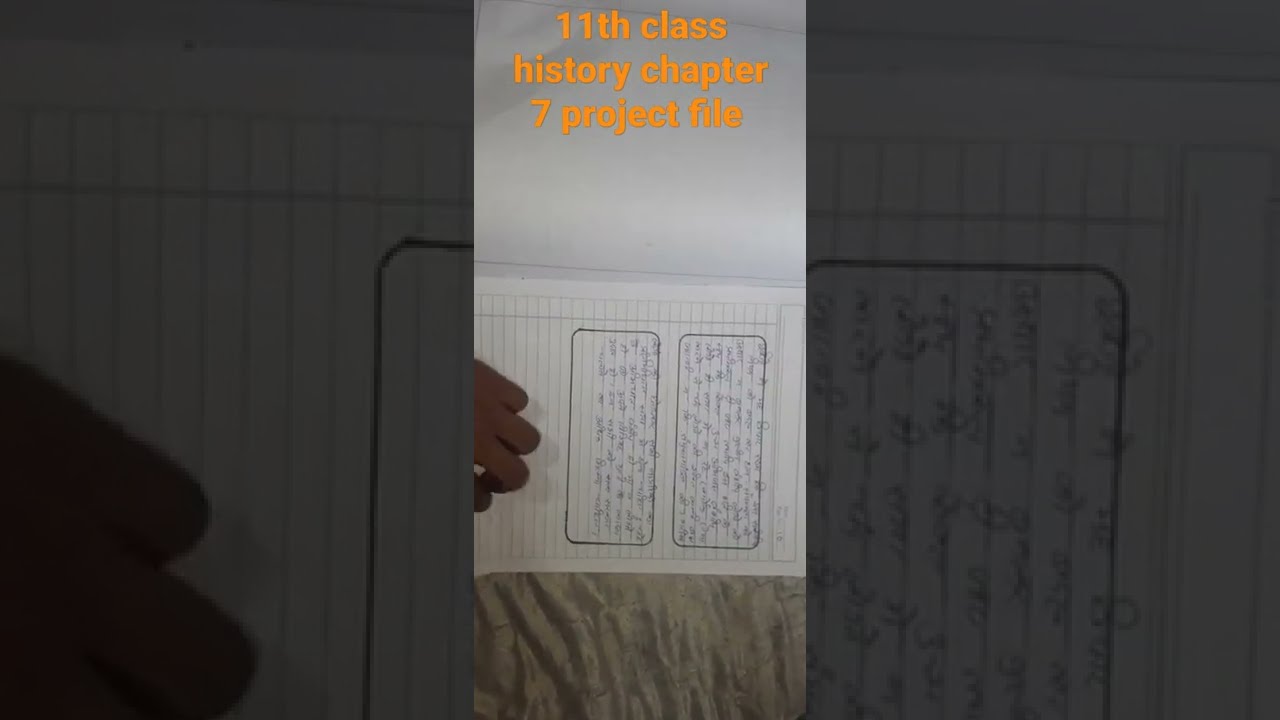This is a horizontally oriented rectangular image featuring a central photograph flanked by large, grayed-out areas on either side. The focal point is a piece of lined paper, likely part of a notebook or binder, which is lying flat on a tan bedspread with a white wall in the background. The paper is positioned sideways, displaying text that is difficult to decipher from this distance but is written in cursive, possibly in blue ink. There are two black-pen drawn boxes on the paper, each containing a paragraph of text. A brown, illustrated hand with three fingers and a thumb can be seen at the bottom of the paper, adding an animated touch to the scene. Prominent orange text at the top of the photograph reads, "11th Class History Chapter 7 Project File." The image is layered, with the central photograph highlighted and the side areas showing zoomed-in, partially obscured portions of the same lined paper, emphasizing the main content in the middle.